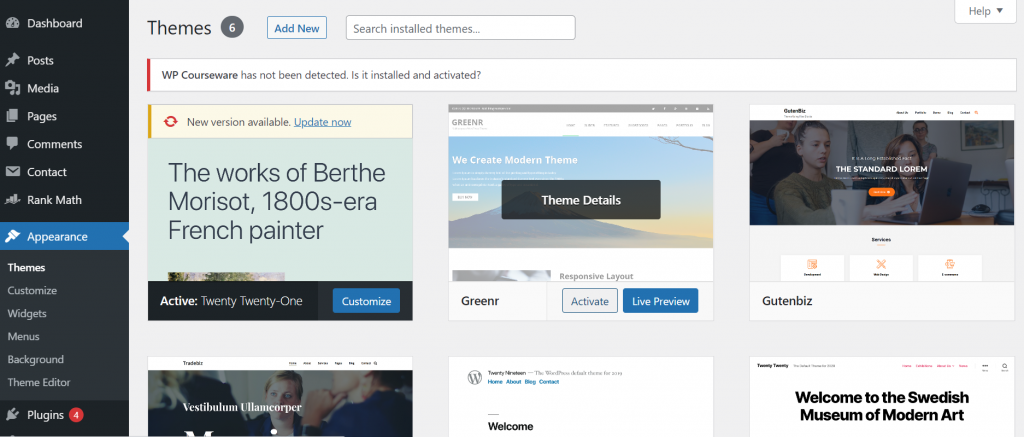The image is a detailed screenshot of a website theme selection interface, likely part of a website building tool. On the far right, there is a tall, rectangular gray sidebar featuring several icons accompanied by descriptive text options. The icons start with a dashboard icon labeled "Dashboard" at the very top, followed by a pushpin icon with "Posts," a camera icon with two music notes labeled "Media," two overlapping pages with "Pages," a speech bubble with "Comments," and an envelope with "Contact." Additionally, there is a graph icon labeled "Rank Math," and next, a paintbrush icon highlighted in blue labeled "Appearance." Below this, under "Appearance," the subsections "Themes," "Customize," "Widgets," "Menus," "Background," and "Theme Editor" are listed in white letters, with the latter options in a lighter shade indicating they are less prominently featured. Beneath these, a darker gray area is labeled "Plugins," showing a red circle with a white number '4' indicating pending updates or notifications.

The central and left portions of the image dominate with a theme selection interface. At the top left, in gray letters, is the word "Themes." Adjacent is a gray circle with the number '6' inside, followed by a red and blue button labeled "Add New," and a long white text box for searching installed themes. In the upper right corner, there's a "Help" box with a small down-facing triangle.

Below these, the interface displays three main theme options. The leftmost theme features a large beige box titled "New Version Available," with a golden bar beside a red refresh icon. A blue hyperlink states "Update Now," with a light blue description below reading "The works of Berthe Morisot," referencing the 1800s French painter. Part of a painting is visible in the lower left, beneath a black bar reading "Active 2021." To the right is a blue "Customize" box.

The middle theme showcases a faint image of nature with a gray box in the center labeled "Theme Details." Below it, blue boxes labeled "Activate" and "Live Preview" appear, relating to the theme named "GreenR." Smaller boxes with options and icons are also visible.

The rightmost theme presents a grayscale image of two women working at a laptop, labeled "Standard Lorem" in white letters. Additional text appears too small to read, with "Gunt Biz" in black letters at the bottom left.

At the image's bottom, three partially visible theme choices are cut off. The leftmost shows several business attire-clad individuals, only leaving discernible that the accompanying text is in a foreign language. The center theme features a WordPress logo with illegible black, gray, and blue text and the word "Welcome" in black. The theme on the right displays "Welcome to the Swedish Museum of Modern Art" in black letters, with additional text too small to read.